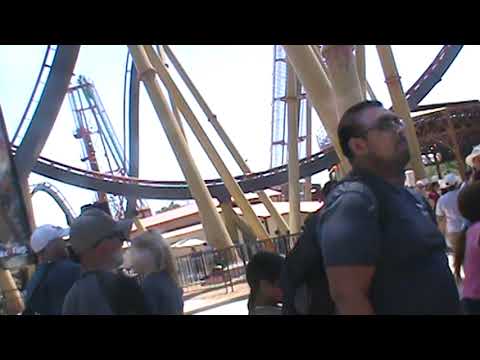The square image captures a bustling scene at an amusement park. In the immediate foreground, several people are noticeable: a large, muscular man in a dark polo or t-shirt on the bottom right, a blonde-haired woman in a dark top conversing with two gentlemen wearing baseball caps on the bottom left, and a young boy possibly waiting in line. Dominating the bottom right is a man with a backpack, dressed in a blue polo shirt and glasses. The background is filled with the intricate, metallic structures of amusement park rides, including a prominent blue loop and yellow supporting poles from a roller coaster. Beyond the rides, there’s a hint of a food court area, indicated by umbrellas and blurred faces of patrons enjoying the sunny day. The pale blue sky adds to the bright, joyful atmosphere, suggesting a perfect day out at the park.